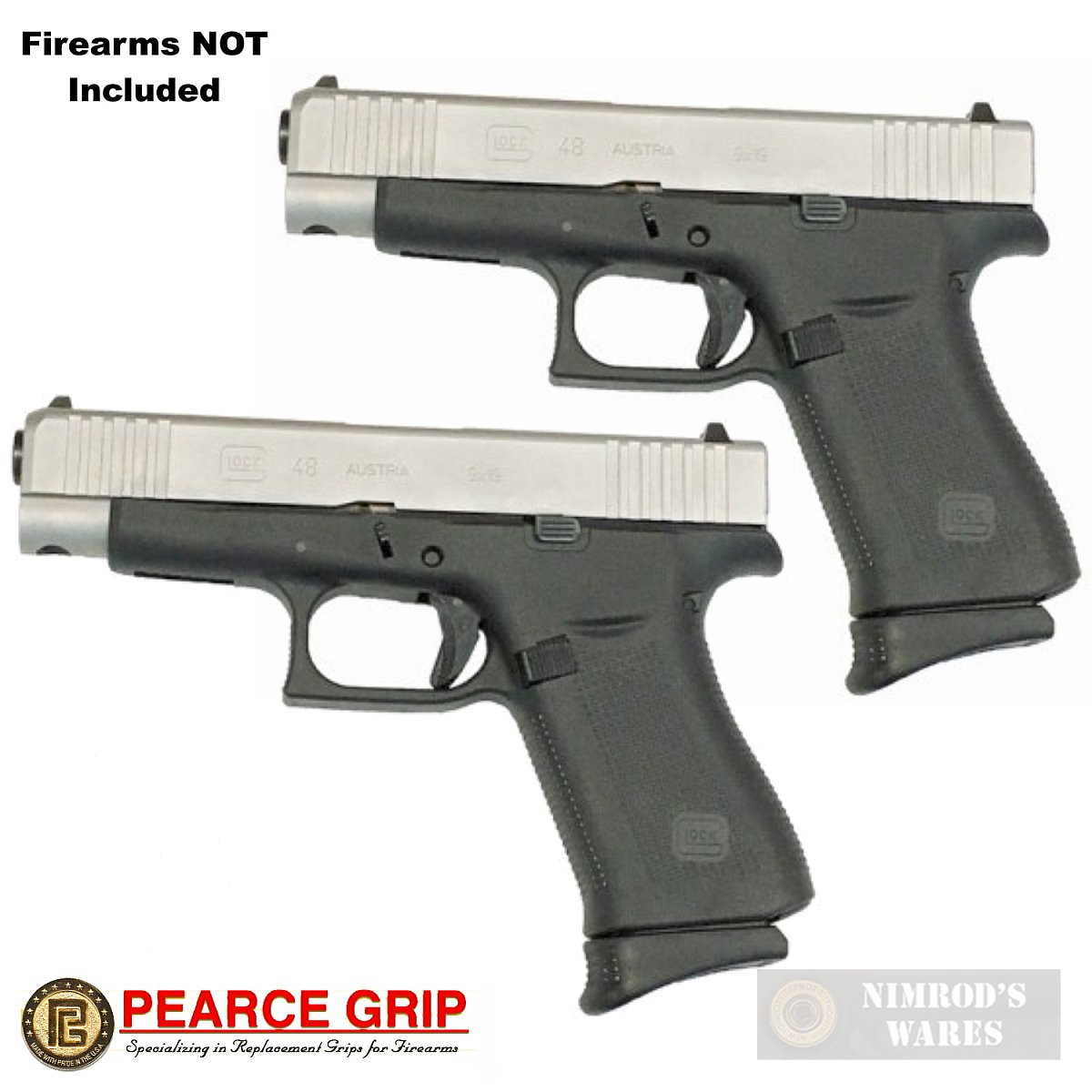The image features two Glock handguns set against a white background. Both guns possess black handles, triggers, and trigger guards, with distinct silver slides on top. Visible on the slides are the inscriptions "48" and "Austria," along with the Glock logo stamped into the metal. The handguns each have a magazine attached at the bottom. In the upper left corner, the text "Firearms Not Included" is displayed. The bottom left corner features the Pierce Grip logo, a coin-shaped emblem with initials "P" and "G," accompanied by the text "Pierce Grip specializing in replacement grips for firearms." The bottom right corner bears a faint watermark-like inscription reading "Nimrod's Wares," with a small bullet icon to the left of the text.